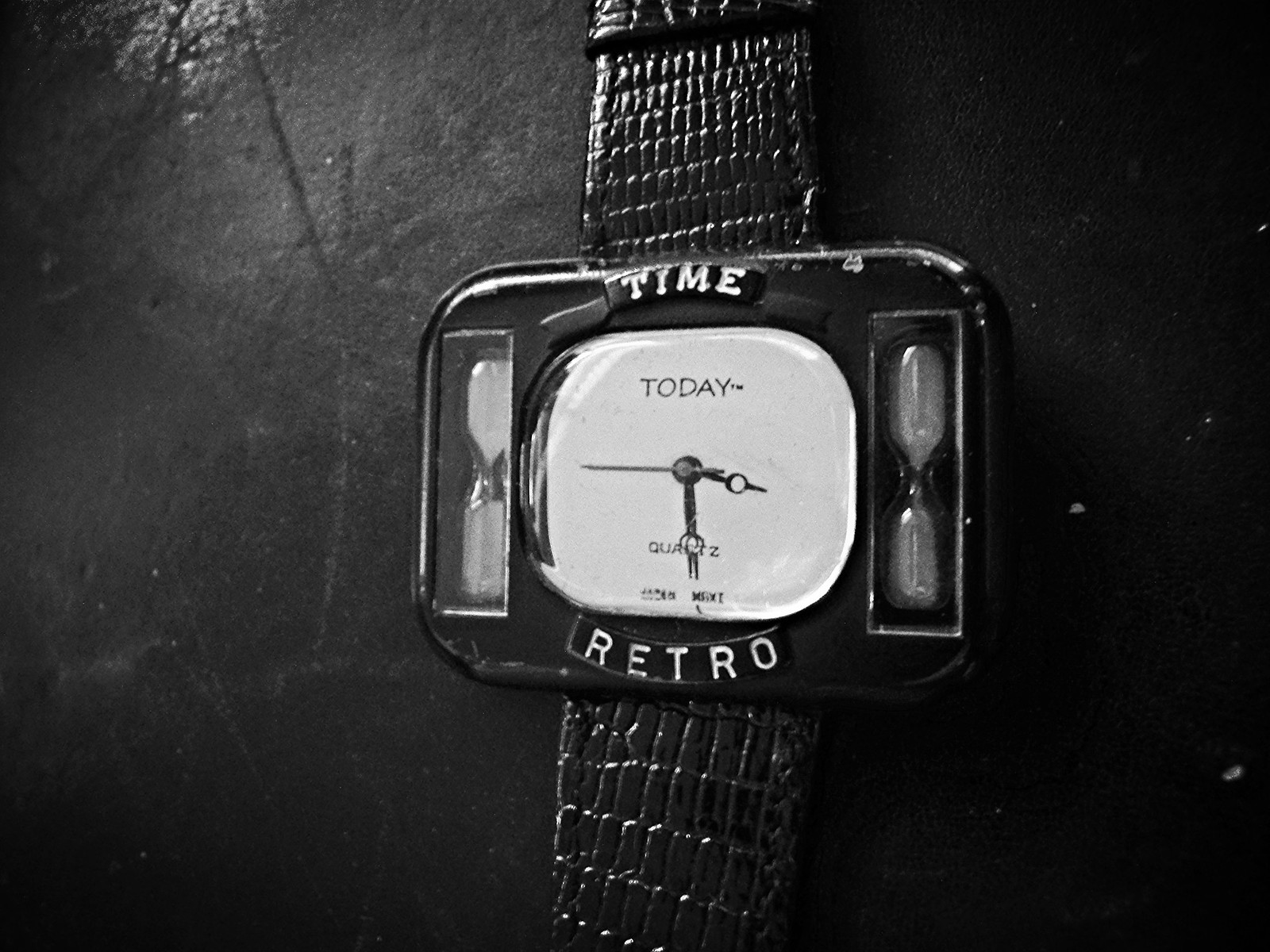A meticulously detailed black and white photograph showcases a unique wristwatch. The face of the watch features a large triangle design, incorporating a central square with rounded corners that serves as the clock face itself, characterized by its clean, white coloration. The clock face is flanked by what appear to be hourglasses set into the black plastic frame; these hourglasses are transparent and may be made either of glass or plastic, containing something white inside.

The design elements include the word "TIME" in white lettering positioned above the clock face and the word "RETRO" also in white, situated below. The face of the clock prominently displays the word "TODAY" in black lettering at the top, while the term "QUARTZ" is visible beneath the hands. There's additional, very small text that's unreadable due to its size. 

Notably, the clock face omits numerical markers, instead featuring plain black hands with a distinctive design: each hand has a black circle with a cut-out section, revealing the background through the middle. The hands are positioned at approximately 4:30. The wristwatch strap resembles an alligator texture, adding to the sense of vintage elegance, all set against a solid black background that enhances the watch's striking appearance.